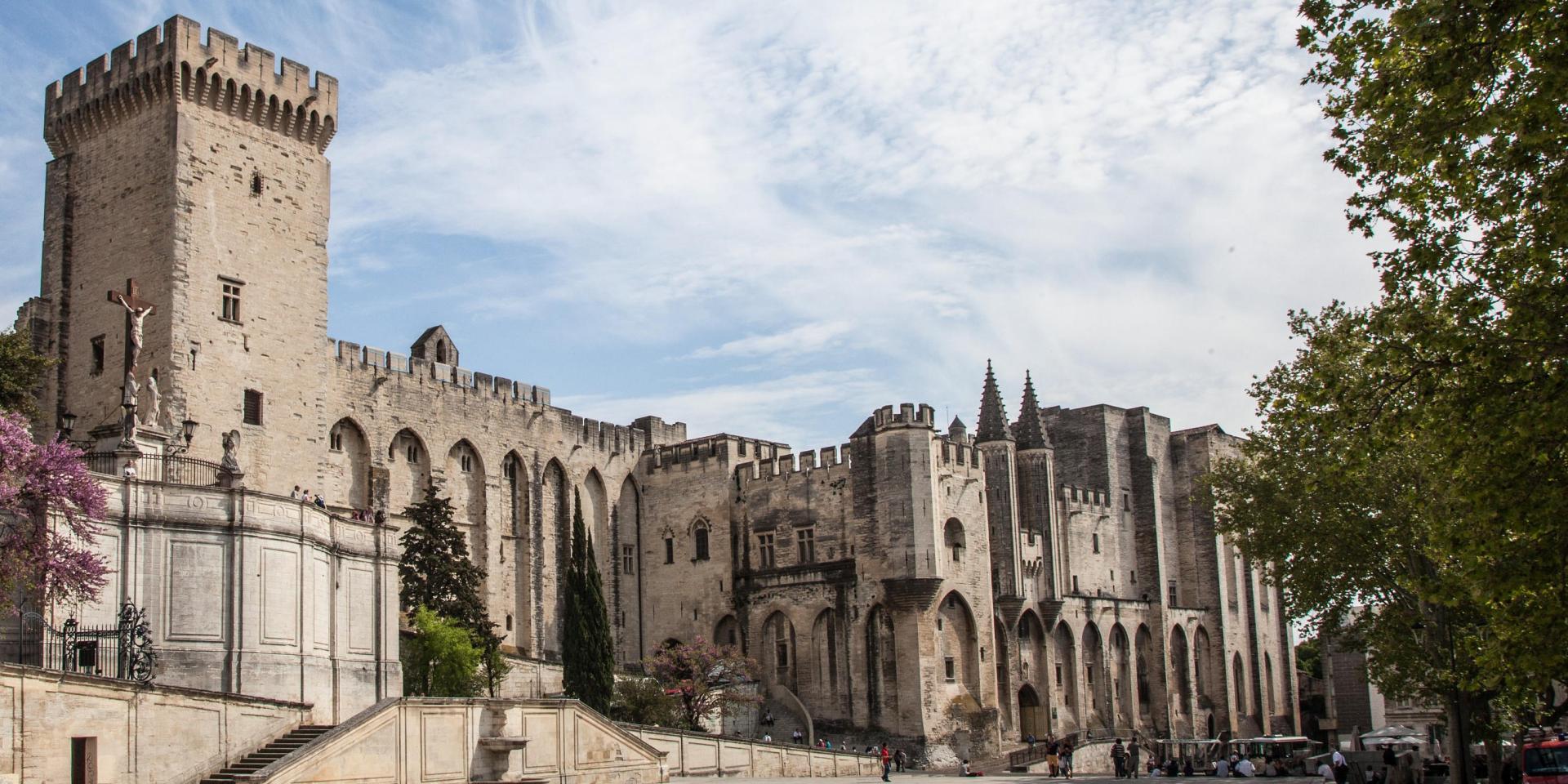The photograph captures a stunning historic building, primarily resembling a large, ancient castle or cathedral, constructed from stone. Dominating the sky with its grandeur, the structure boasts numerous steep roofs, tall towers, turrets, and castellated parapets. The building features several arched walkways and domed windows that contribute to its medieval charm. The left side of the image highlights a square tower while the structure tapers off to the right with additional ornate elements such as tall arches and battlements.

A significant focal point includes a large crucifix statue of Jesus Christ, positioned on the left side near one of the towers. This detail suggests a religious significance, possibly indicating part of the structure serves as a church or cathedral. The sky above is a mix of blue and white clouds, lending a slightly overcast but bright feel to the scene. Trees of varied types, including evergreens and one with striking pink blossoms, frame the building and hint at a landscaped courtyard.

In the foreground, numerous people are visible, indicating the location is a popular tourist spot. Structural details such as stone stairways provide access around the building, and a small tree with pink flowers adds a touch of softness to the otherwise robust stone architecture. The whole scene is enveloped in a hazy, sunny atmosphere that casts gentle shadows, further accentuating the size and ancient beauty of the castle-like edifice.